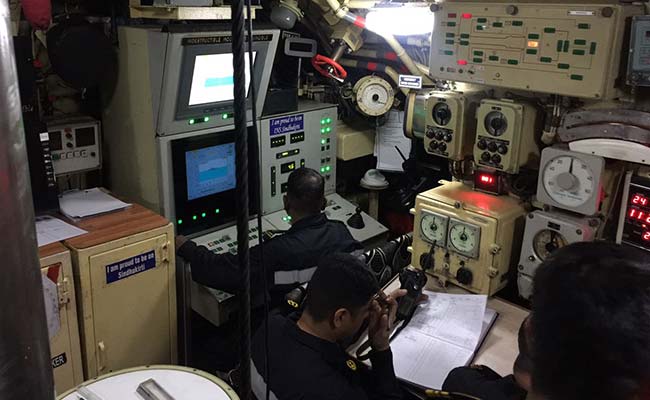This photograph captures an indoor scene resembling a mission control room or a submarine control room, filled with an array of electronic equipment and surrounded by various devices and gauges. At the bottom center of the image, two men are sitting at different workstations. The man closest to the viewer, dressed in a black jumpsuit with a reflective silver stripe on the back, is sitting at a desk facing to the right. In front of him is a paper log sheet, and he is scratching his forehead with a pen. Behind him, another man, likely a black man, is engaged with a computer terminal that features a screen, numerous buttons, and a joystick.

The walls are adorned with numerous electronic boxes, varying in size and type. Some of these boxes are square with dials and black knobs, while others are rectangular with dials, knobs, and control panels. Prominently, there are large rectangular boxes with green, red, and white lights and diagrams. The equipment comes in shades of gray, silver, cream, and beige. On the right-hand side of the room, a man is holding a walkie-talkie with papers in front of him. On the left, another man sits amidst silver equipment bearing green lit buttons and an additional screen positioned above his computer monitor. Overall, the room is cramped but meticulously equipped, exuding an atmosphere of high-stakes operations.